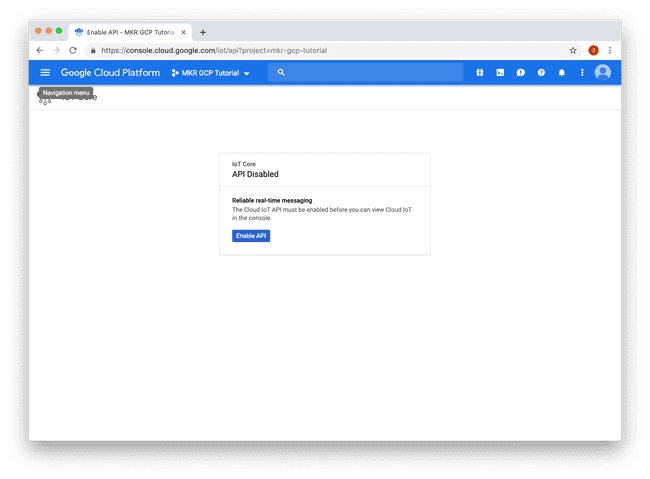Screenshot of the Google Cloud Platform Console displayed on a computer screen, likely from a laptop or desktop using the Google Chrome browser, as indicated by the position of the tabs' close (X) buttons on the right side of the interface. The visible webpage is the Google Cloud Console, specifically showing a notification within the Cloud IoT (Internet of Things) Core section. A dialog box prominently positioned in the center of the screen alerts the user that the "Cloud IoT Core API is disabled" and includes a message about enabling it for reliable real-time messaging capabilities. The page is minimalistic with a clean layout dominated by a white background and a blue navigation bar at the top. This stark interface underscores functionality over aesthetics, likely aimed at users with IT or technical expertise, providing essential information without unnecessary visual clutter.